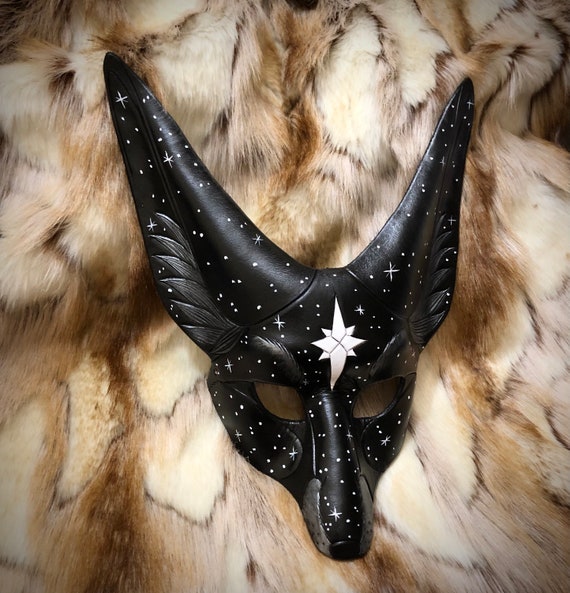The image displays a striking black mask designed in the shape of a fox, featuring tall, pointed ears and small eye holes that are blank. The mask is adorned with numerous small stars and white specks, with a prominent, large white star positioned between the eyes on the forehead. The snout area is distinctly shaped, adding to the fox-like appearance. The mask is set against a plush fur background, which appears to be a fur rug or coat in shades of tan, white, and brown, with some black lines or streaks throughout. The detailed starry motif on the mask contrasts with the soft, textured fur, creating a unique and visually intriguing composition.